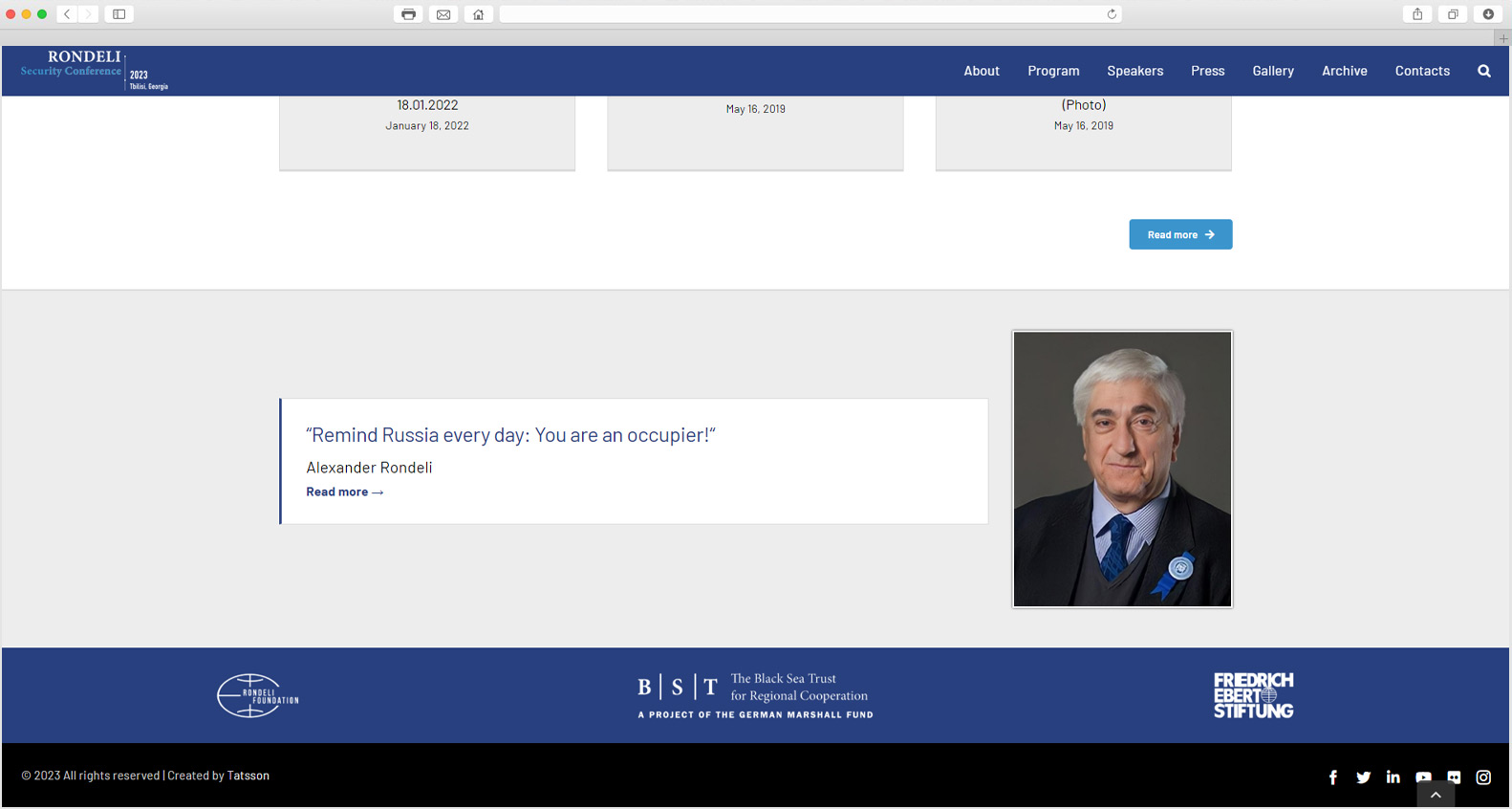At the Rondelli Security Conference 2023 in Tbilisi, Georgia, the screen displays a detailed layout dominated by a prominent blue bar across the top. On the left side of this bar, the text reads "Rondelli Security Conference," followed by "2023 in Tbilisi, Georgia." Also on the left, neatly arranged are navigation options: About, Program, Speech, Press, Gallery, Archive, and Contacts.

As the screen scrolls down, partial views of several content boxes become visible, each labeled with different dates—January 18, 2022, coinciding with an entry labeled "Photo, May 16, 2019."

Dominating the lower half of the very wide screen is mostly blank space, punctuated by a blue box towards the right that reads "Read More" with an arrow pointing to the right. Beneath this, in a large ivory off-white box, stands an image of an older man with silver hair, dressed in a full suit and adorned with a star ribbon badge on his lapel. Beside his picture runs a striking quote: "Remind Russia every day, you are an occupier!" attributed to Alexander Rondelli, inferred to be the person in the photograph.

Below this, a navy blue box outlines an important note: "The Black Sea Trust Regional Cooperation, a project for the German Marshall Fund," alongside "Friedrich Ebert Stiftung."

Concluding the layout at the bottom, a black box houses social media icons for Facebook, Twitter, LinkedIn (denoted by IN), Instagram, and possibly other platforms, providing easy access to various social media channels.